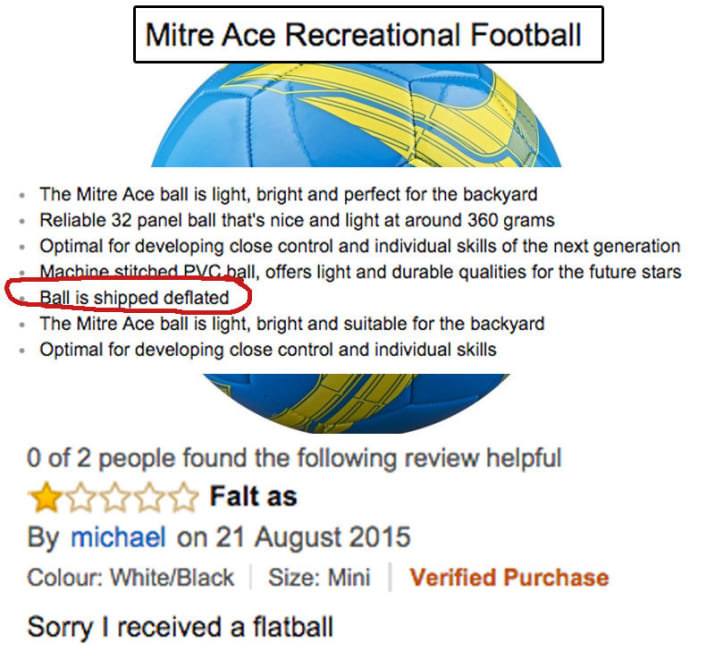This is an older screenshot featuring a product review for the Mitre Ace Recreational Football. At the top, within a white rectangular bar, the product name "Mitre Ace Recreational Football" is written in black text. Below, a larger white bar with seven bullet points overlaps a drawing of the football, which is blue with yellow designs.

**Bullet Points:**
1. The Mitre Ace Ball is light, bright, and perfect for the backyard.
2. Reliable 32-panel ball that's nice and light at around 360 grams.
3. Optimal for developing close control and individual skills in the next generation.
4. Machine-stitched PVC ball offers light and durable qualities for future stars.
5. The statement "Ball is shifty flated" is highlighted with a red circle around it.
6. The Mitre Ace Ball is light, bright, and suitable for backyard use, and optimal for developing close control and individual skills.

Below the bullet points, there is a review. Zero out of two people found the review helpful. The review shows five stars, but only one star is highlighted. 

**Review Details:**
- Reviewer: Michael
- Review Date: 21 August 2015
- Color: White/Black
- Size: Mini
- Purchase: Verified
- Review Text: "Sorry, I received a flat ball."